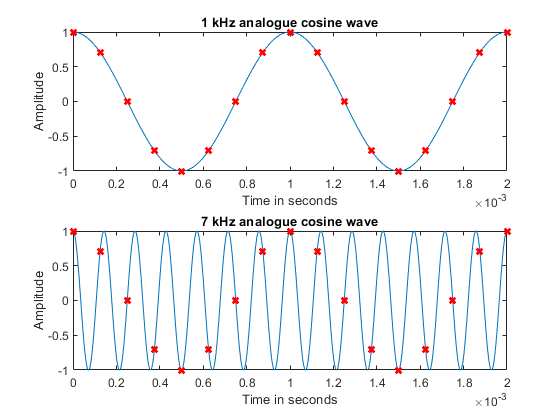The image showcases two distinct graphs on a white background, each highlighting different frequency cosine waves. Both graphs share the same axes: the y-axis labeled "Amplitude" ranging from -1 to 1 in 0.5 increments, and the x-axis labeled "Time (in seconds)" extending from 0 to 2 in 0.2 increments. The top graph illustrates a "1 kHz Analog Cosine Wave," depicted by a blue sinusoidal line starting from the top left, creating a few gentle humps along its course. Red X marks are scattered along the wave, indicating specific points. The bottom graph displays a "7 kHz Analog Cosine Wave," where the blue wave oscillates far more frequently, appearing much tighter and denser compared to the top one. Here again, red X marks are placed at various intervals along the wave.